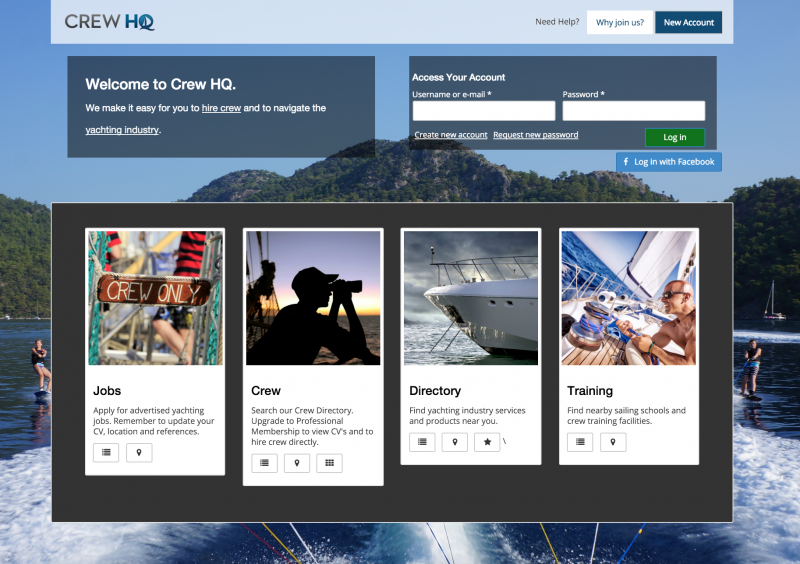The image depicts a picturesque scene with a body of water in the background. Several individuals are engaging in water sports, possibly water skiing or surfing, and are connected by tow lines to an unseen source off the image. A majestic mountain and a clear blue sky provide a stunning backdrop.

At the top of the image, bold text reads "Crew HQ," followed by a welcoming message: "Welcome to Crew HQ. We make it easy for you to hire crew and to navigate the yachting industry." To the right, there are fields for users to access their accounts, with input boxes labeled "Username or Email" and "Password."

Below this, a black box features four sections, each with distinct details:
1. The first section, labeled "Jobs," includes an image with "Crew Only" and a prompt encouraging users to apply for advertised yachting jobs. It reminds users to update their CV, location, and references.
2. The second section, labeled "Crew," shows a silhouette of a person using binoculars on the ocean and invites users to search the crew directory. It mentions the option to upgrade to professional membership to view CVs and hire crew directly.
3. The third section, labeled "Directory," depicts a boat on the ocean and guides users to find yachting industry services and products near them.
4. The fourth and final section, labeled "Training," features an image of a man tying something down on a boat and directs users to find nearby sailing schools and crew training facilities.